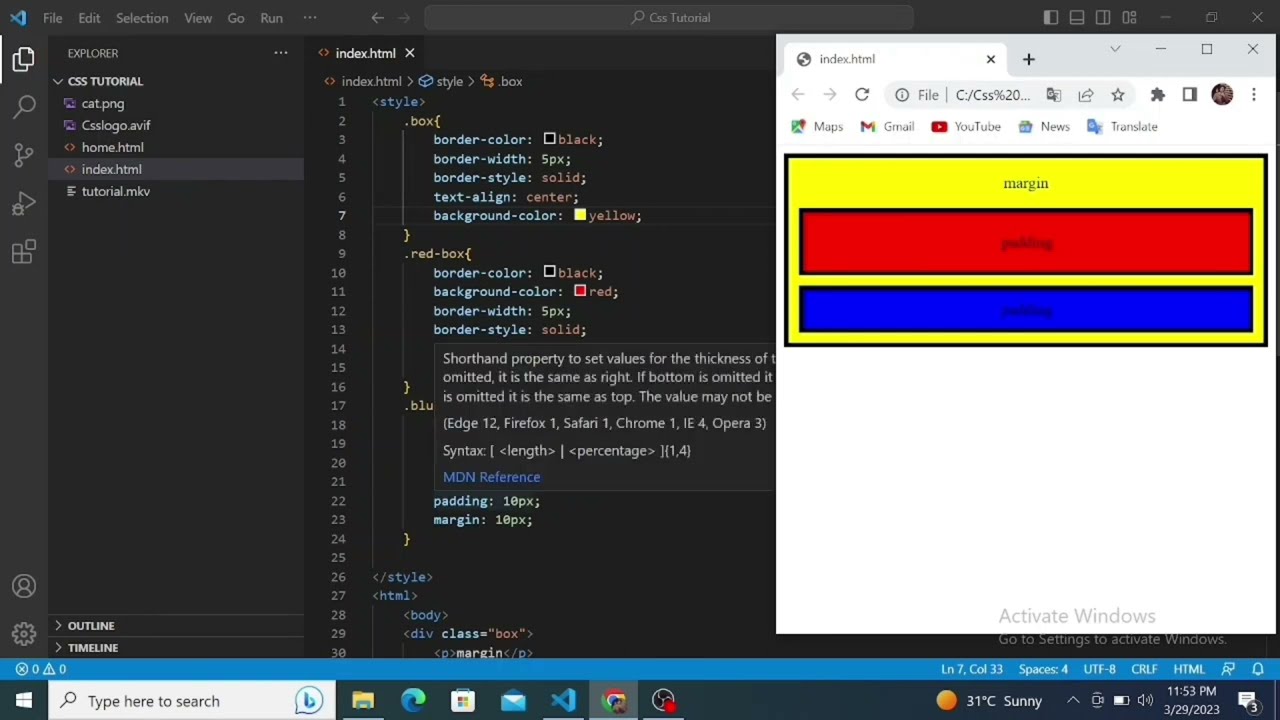This image captures a detailed screenshot of a computer screen, showcasing a coding environment for a CSS tutorial. The interface is predominantly dark, featuring a black background. On the far left, a column displays an open folder labeled "CSS Tutorial," with a series of subfolders beneath it, and an explorer icon above. To the right is an active tab named "Index.html," displaying lines of HTML code divided into four sections, including a paragraph discussing shorthand property for border thickness.

Above the coding area, the header menu in light gray print reads: File, Edit, Selection, View, Go, Run, along with a magnifying glass icon labeled "CSS Tutorial." Adjacent to this coding section, a white pop-up window appears with a header showcasing icons for Maps, Gmail, YouTube, and News. Directly within this window is a yellow rectangle with a black outline, titled "Margin." Inside the yellow box are two rectangular buttons, one red and one blue, although their text is blurred and unreadable. At the bottom of the screen, a footer bar includes a search bar, folder tabs, mail icons, weather details indicating 31 degrees and sunny, and a clock displaying 11:53 PM. This comprehensive setup strongly indicates a detailed tutorial or a coding class environment.